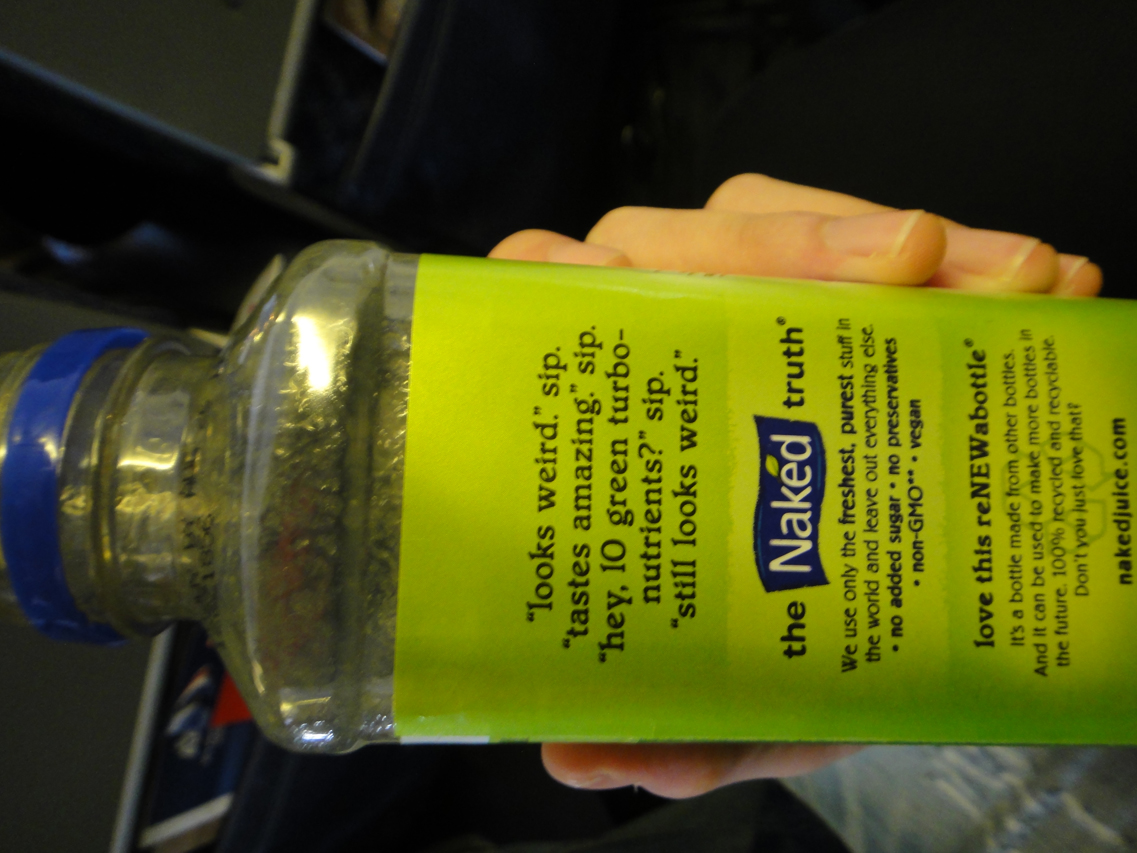In this rectangular photograph, we observe a hand holding a bottle in a sideways position. The hand, characterized by Caucasian skin tone, displays the thumb at the bottom and the four fingertips gripping the top. The bottle, adorned with a light green label, features an open mouth sealed with blue plastic. The label contains various inscriptions in black text, reading: "The naked truth. Looks weird, sip. Tastes amazing, sip. Hey, 10 green turbo nutrients, sip. Still looks weird. Interesting label." Further down, it elaborates, "We use only the freshest, purest stuff in the world and leave out everything else. No added sugar, no preservatives, non-GMO, and vegan. Love this Renew bottle." The label also includes the brand's website, NakedJuice.com. The image highlights the unique and health-conscious branding of the Naked Juice bottle being presented by a human hand.